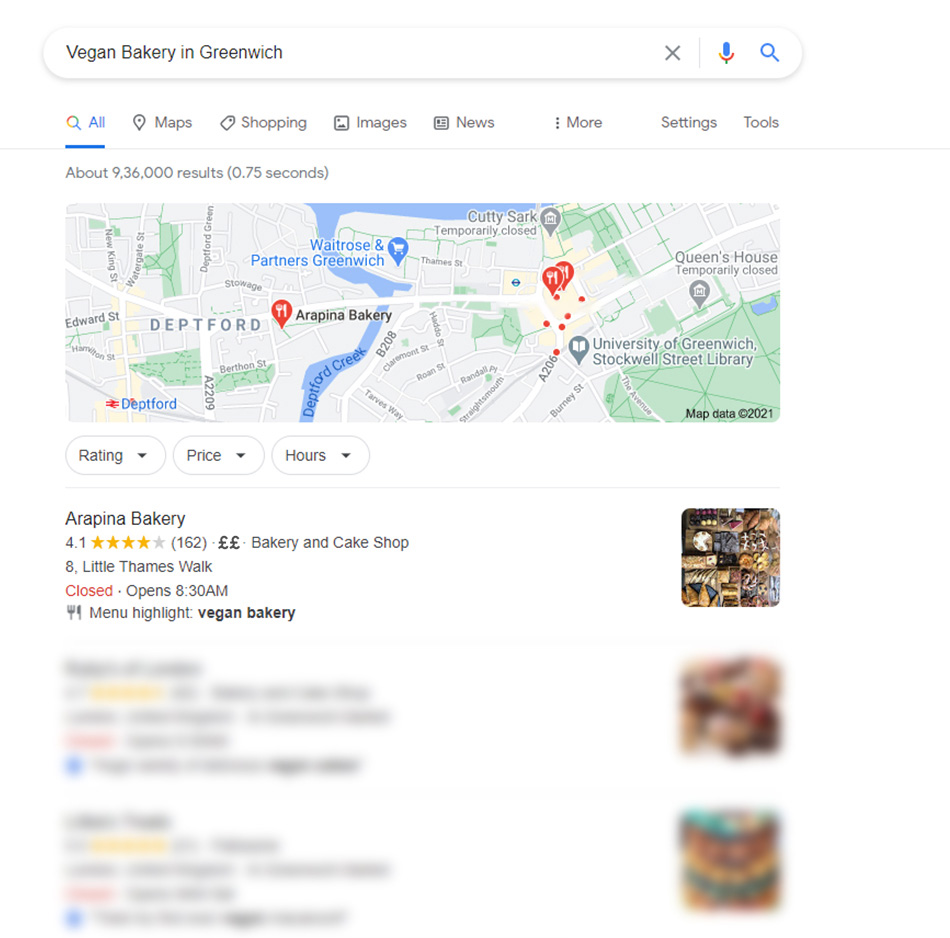The image displays a web browser with an open search query for "vegan bakery in Greenwich." The search term is prominently shown in a white text box with black text, accompanied by a small black "X" on the right side of the box. Adjacent to the text box, there are blue icons for a microphone and a magnifying glass symbolizing voice search and search functionality, respectively.

At the top of the browser, there is a navigation bar with gray text links for various categories, including "All," "Maps," "Shopping," "Images," "News," "More," "Settings," and "Tools." Directly below this navigation bar, a map is displayed with several red markers indicating locations of interest. The map also features roads and a blue waterway labeled "Deptford Creek."

Below the map, the search results list begins with Arapena Bakery, which has an accompanying rating of 4 out of 5 stars, based on 162 reviews. To the right of this information is a photograph depicting the interior of the bakery, showcasing an array of breads and other food items. The top search result is highlighted in red, indicating that the bakery is currently closed.

There are two additional search results visible, but they appear to be blurred out, making the details indiscernible.